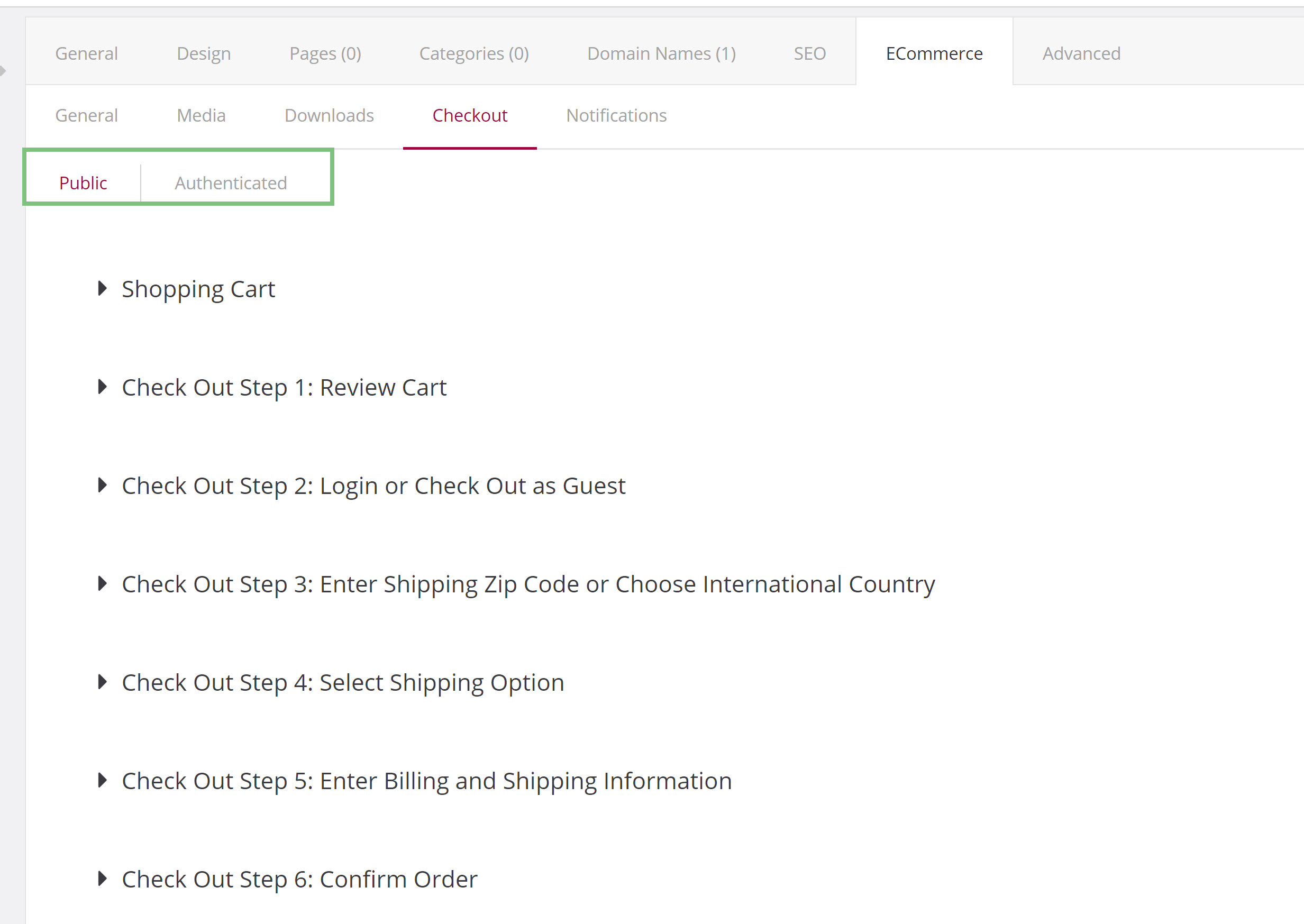The screenshot showcases a webpage with a detailed navigation structure. At the top, the visible tabs read from left to right: "General Design Pages" (0), "Categories" (0), "Domain Name" (1), "SEQ," "E-Commerce" (highlighted), and "Advanced." Under the highlighted "E-Commerce" tab, a subcategory menu is displayed with the following options: "General," "Media," "Clouds," "Checkout," and "Notifications," with "Checkout" being the highlighted option. This selection reveals additional categories named "Public" and "Authenticated," where "Public" is highlighted and "Authenticated" is grayed out. The "Public" category further expands into a detailed list of checkout steps, including "Shopping Cart," "Checkout Step 1: Review Cart," "Checkout Step 2: Log In or Checkout as Guest," "Checkout Step 3: Enter Shipping Zip Code or Choose International Country," "Checkout Step 4: Select Shipping Option," "Checkout Step 5: Enter Billing and Shipping Information," and "Checkout Step 6: Confirm Order."